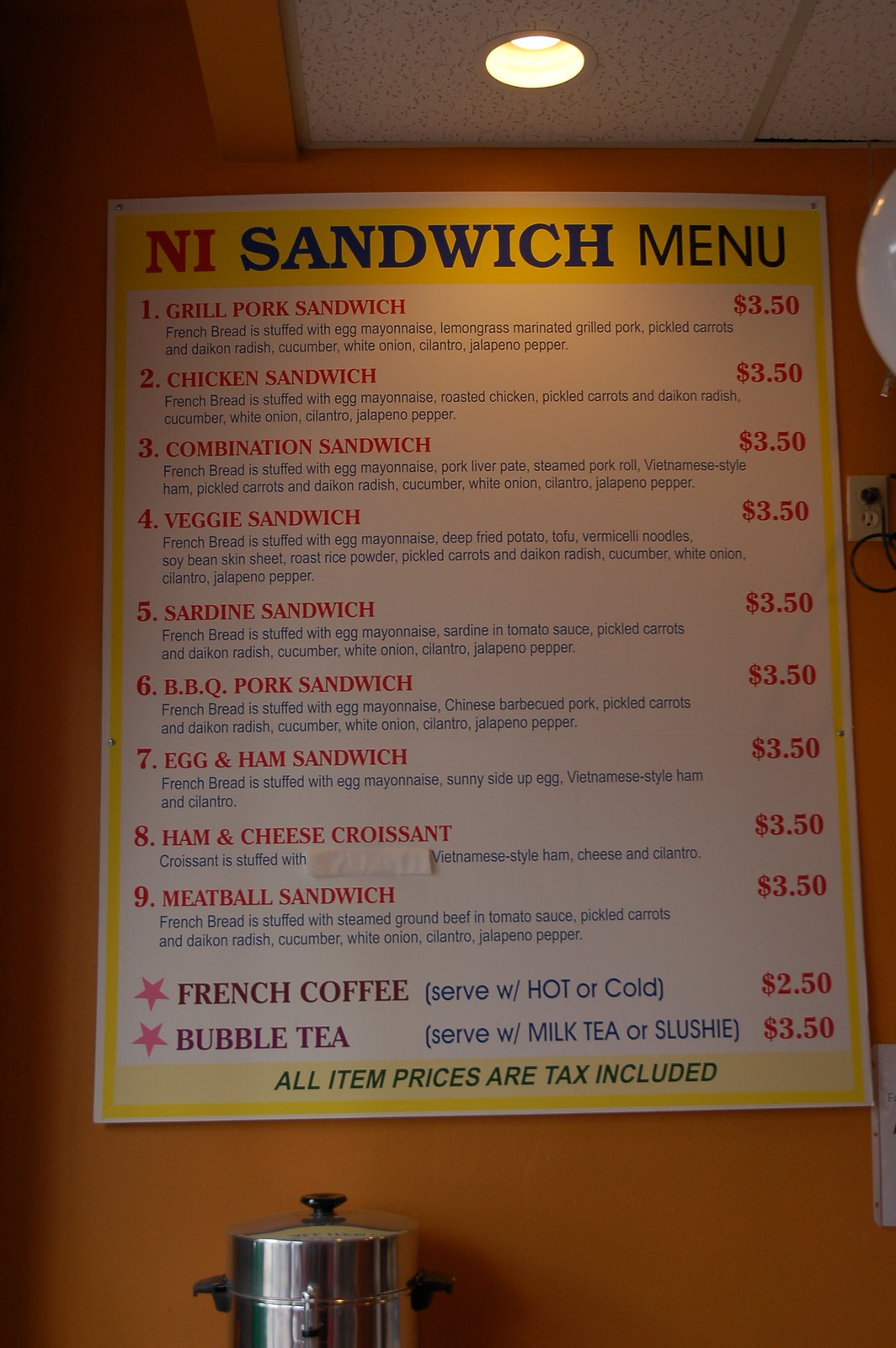The image showcases a vibrant restaurant setting, with a prominently displayed menu mounted on an orange wall. The rectangular menu, designed in a portrait orientation, features a white and yellow background adorned with red and black lettering. The top of the menu reads "NI" in bold red letters, followed by "Sandwich Menu" in black.

The menu lists a selection of sandwiches:

1. Grilled Pork Sandwich
2. Chicken Sandwich
3. Combination Sandwich
4. Veggie Sandwich
5. Sardine Sandwich
6. Barbecue Pork Sandwich
7. Egg and Ham Sandwich
8. Ham and Cheese Sandwich
9. Meatball Sandwich

Additionally, the menu offers beverages such as French Coffee and Bubble Tea, with prices conveniently listed to the right of each item, indicating that all prices include tax.

Beneath the menu, a stainless steel pot is present, likely containing coffee or another hot liquid. To the right of the menu, an electrical socket with a plug can be seen, along with a partially visible large white circle that appears to be a light fixture. There is also a red and white paper object, adding to the eclectic decor of the space. The combination of bright colors and detailed elements creates an inviting atmosphere for patrons.